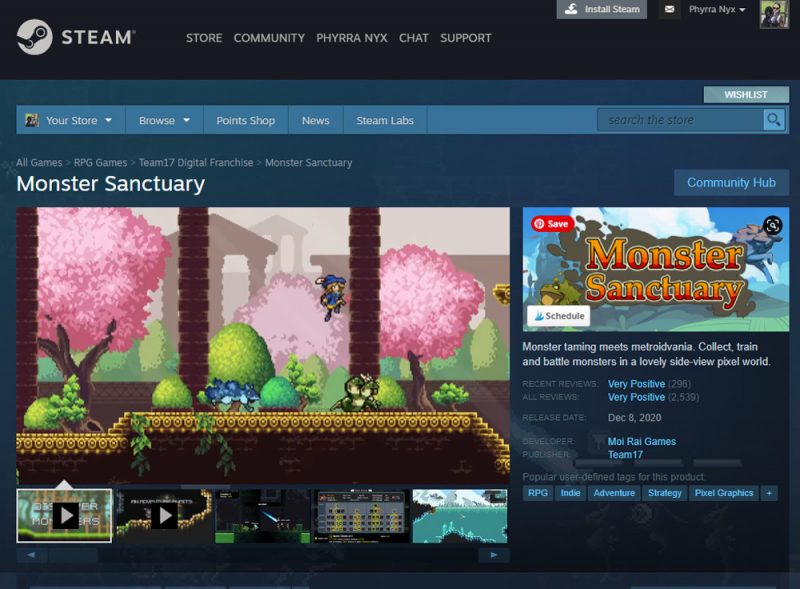This landscape-oriented screenshot appears to be from the Steam gaming platform. At the top of the image, a black horizontal banner spans the width of the screenshot, featuring white text and icons. To the far left, there's a circular icon resembling the face of a putter labeled "STEAM." Following this, clickable links labeled "Store," "Community," "PYHRR," "ANYX," "Chat," and "Support" are displayed.

Beneath the banner, a gray box at the top highlights an "Install Station" button, accompanied by various small, hard-to-read icons. Further down, a blue, horizontally aligned border contains several separated boxes and drop-down menus. The first box showcases an avatar next to the text "Your Store" with a white drop-down menu, followed by "Browse" with another drop-down menu. Neighboring these are options for "Points Shop," "News," "Steam Labs," and a search bar to the right.

Under this bar, a header labeled "Monster Sanctuary" features an image of the game. The game's graphics evoke nostalgia with a style reminiscent of classic Zelda or Mario games, showcasing cherry blossom trees and a character running and jumping. To the right of this image, another graphic with the "Monster Sanctuary" title is displayed against a scenic background, highlighted by red and yellow letters. Above this graphic, a save button is visible.